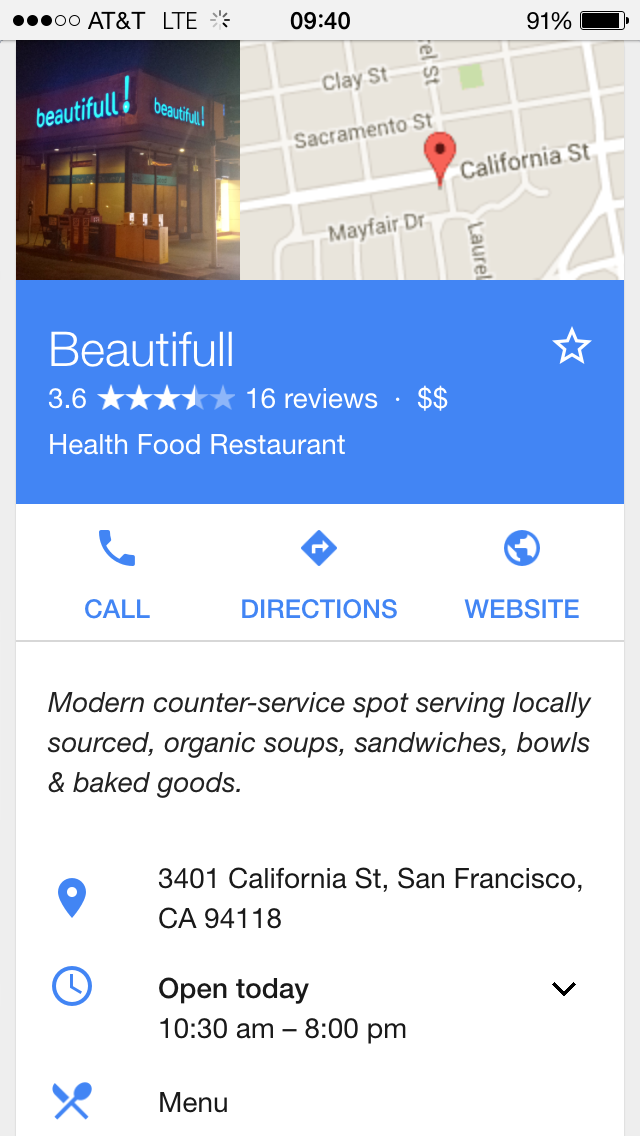Screenshot of Google Maps page for "Beautiful," a health food restaurant, highlighting key details. In the upper right corner, a small map pinpoints its location at 3401 California Street, San Francisco, California 94118. The upper left corner shows a picture of the restaurant, a square gray building adorned with the word "BEAUTIFULL!" in neon blue letters on two sides. 

The restaurant's profile indicates it has a rating of 3.6 stars out of 5, based on 16 reviews, and is categorized as moderately expensive, marked by two dollar signs ($$). It is described as a health food restaurant. 

Below, interactive buttons allow users to call the restaurant, get directions, or visit the restaurant's website. 

Further down, a concise description characterizes Beautiful as a modern counter-service spot that serves locally-sourced organic soups, sandwiches, bowls, and baked goods. The establishment's operating hours are from 10:30 a.m. to 8:00 p.m., and there is an option to view its menu.